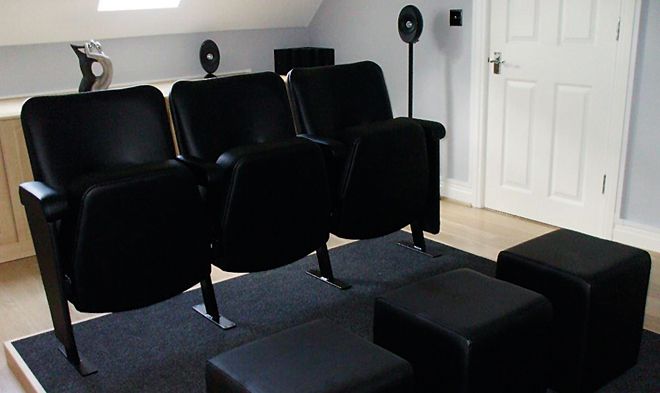The image depicts a small, home theater setup with three black, stadium-style chairs. These chairs are positioned on a raised, black carpeted platform, with their bottoms folded up, resembling typical theater or stadium seating. In front of each chair is a black, cushioned footrest. The room's walls appear to be light blue, and a white door with a silver doorknob is visible on the right side. Behind the chairs, there is a partial view of a window and some decorative elements that look like sculptures or artwork, possibly including black and silver pieces. The floor beyond the platform is a light wood color and slightly blurry. The setup suggests a cozy, personal space for watching movies, enhanced by a light from outside indicating daytime.